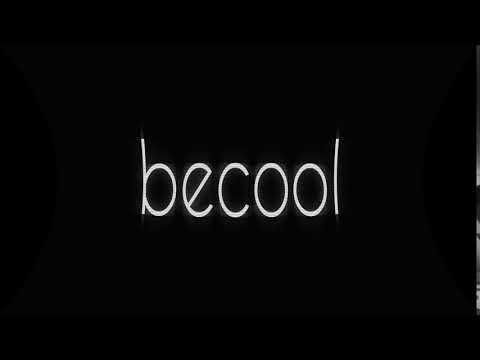The image features a distinctive, contemporary design with the word "BeCool" written in a modern, eye-catching font. The text is in sleek, white letters, without any spaces between the words, against a solid black background. The font is particularly notable for its modern feel, with a uniquely slanted "E" that adds to its appeal. The image is minimalistic, containing no additional elements or text except for a barely noticeable thin strip on the right side, which appears to be a fragment of a black and white photo. This strip is so subtle that it can easily be overlooked at a quick glance, suggesting the image may be cropped from a larger graphic or panorama. The overall impression is that of a stylish logo, possibly for a fashion brand or clothing line, emphasizing simplicity and modernity.